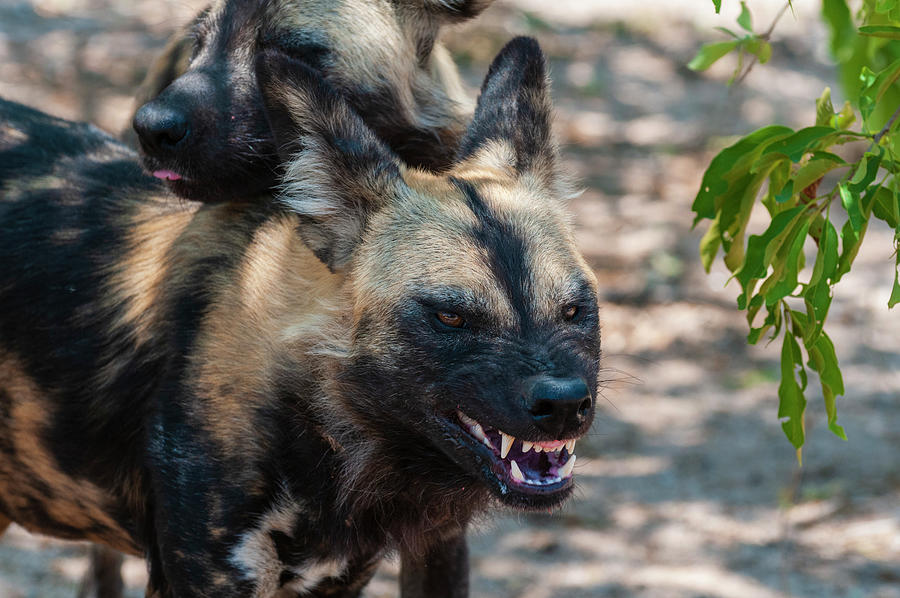This is an image showcasing two wild dog-like mammals outdoors, resembling a cross between a cat and a dog, potentially jackals. The focal animal has a vicious appearance with light tan and black fur, and distinct black markings: a stripe down its two large, pointed ears and a black muzzle. Its sharp, prominently displayed teeth are visible through its open mouth, revealing sharp canines, complementing its slightly scrunched brown eyes, giving it an aggressive demeanor. Resting its head on the back of the first animal is a second one of the same species, appearing more at ease with its tongue slightly sticking out. The scene also includes green leaves to the right and a blurred background with brown and green patches, adding depth to the natural setting.